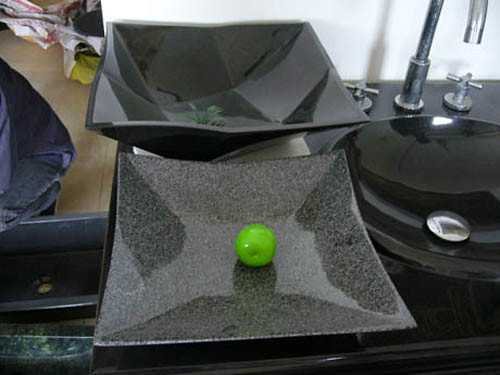The image showcases an intriguing blend of modern and vintage design elements. On the right side, there is a sleek, black counter paired with a black sink featuring a distinctively old-fashioned metal faucet. This juxtaposition creates a striking contrast between contemporary and classic styles. To the left, a sophisticated black plate with a speckled pattern is prominently displayed. At the center of this plate lies a vibrant green object resembling a mini cherry tomato, likely a decorative piece due to its unusually bright hue.

Behind the black plate, a deeper, black container with a conspicuous depth adds another layer of elegance. This modern vessel is accentuated by a minuscule plant positioned at its center, the plant occupying merely 5% of the container's volume, again suggesting a decorative purpose that emphasizes modern minimalism.

The backdrop is a pristine white wall, enhancing the focal points in the image. To the far left, some indistinguishable objects are partially visible, including what appears to be a crumpled piece of paper, adding an element of everyday realism to the otherwise meticulously styled scene.